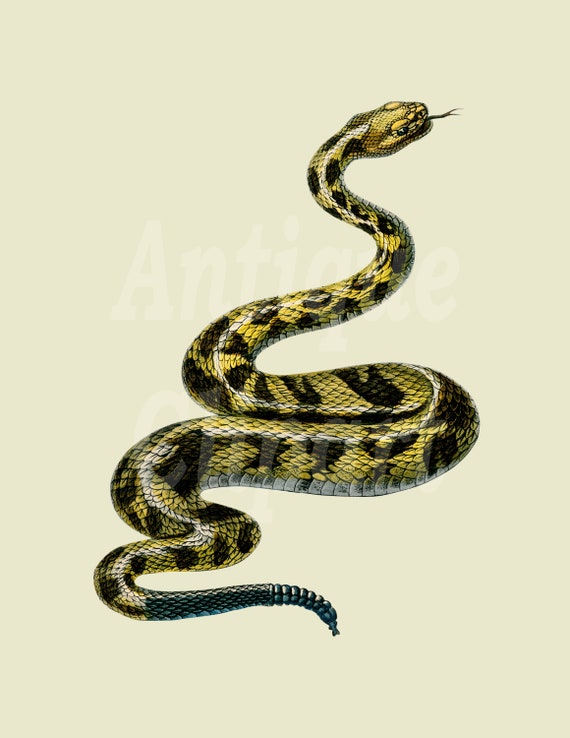The image depicts an illustration of a hissing rattlesnake, prominently positioned in the center with its head angled towards the upper right corner. The snake’s body exhibits a complex series of curls, initially descending downward to the left, then looping sharply to the right and back left before culminating in a blue rattler at the tail end. The snake’s coloration features a mix of yellow and black, with a pattern resembling leopard spots along its body.

The background of the image is a beige, cream-yellow gradient, providing a light contrast to the snake. Superimposed on this background is faint, large text reading "ANTIQUE," with an additional unreadable word beneath it, suggesting a watermark or the author's signature. The image itself is rectangular, approximately six inches high and four inches wide, emphasizing the snake and its striking features against a subdued backdrop.